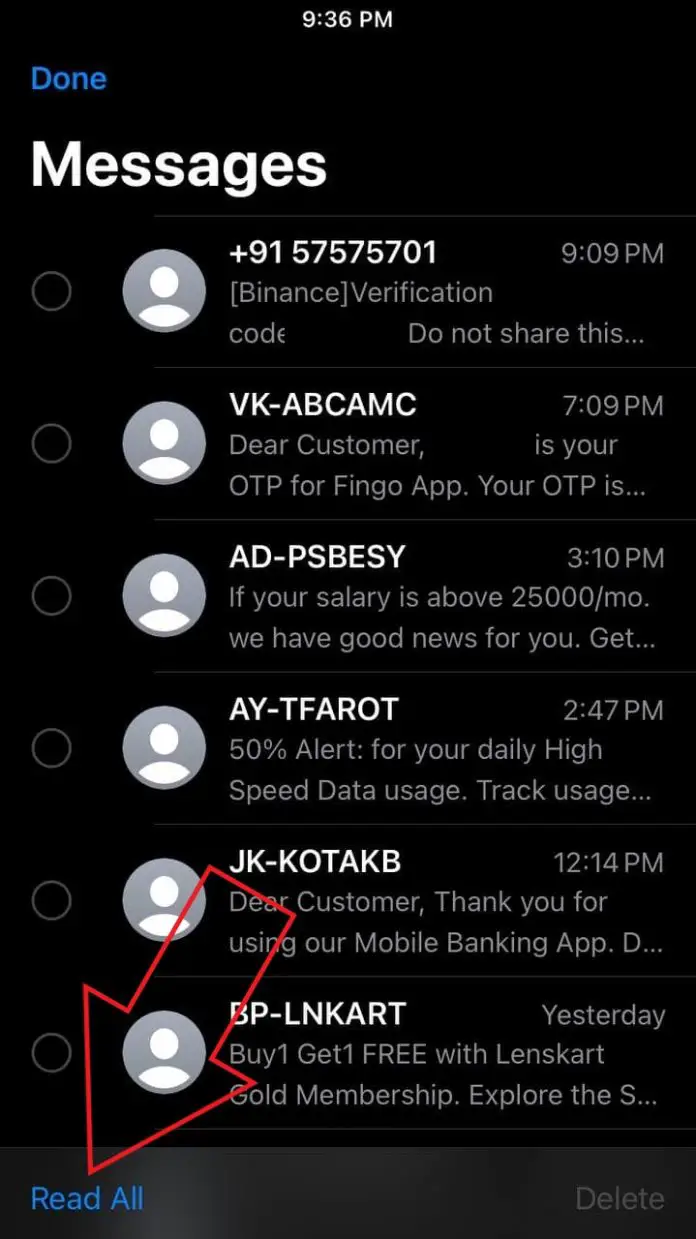The image depicts a screenshot of a mobile phone's inbox, captured at 9:36 PM, as indicated by the white text at the top-center against a black background. The top-left corner features the word "Done" in blue text. Beneath this, the header "Messages" is prominently displayed in large, bold, white font.

The inbox contains about six messages, none of which are highlighted. Each message is marked by a generic avatar—a gray circle with a white silhouette of a person. To the right of these avatars are the contact details of the senders, including:

1. A phone number: +91 575-75-701 at 9:09 PM
2. VK, at 7:09 PM
3. ABC, at 3:10 PM
4. AMC, at 2:47 PM
5. ADPS, at 12:14 PM
6. BESY, timestamped "yesterday"

Each sender has a unique identifier, spanning from alphabetic labels like "VK" to "BPLNKART." The messages' content is briefly mentioned but not detailed in the description.

Located in the lower-left is a downward-pointing arrow outlined in red, directing attention to a "Read All" option in blue text. In the bottom-right corner, a button labeled "Delete" is visible.

This detailed view showcases a variety of message senders, times, and the interface options available to the user for managing their messages.